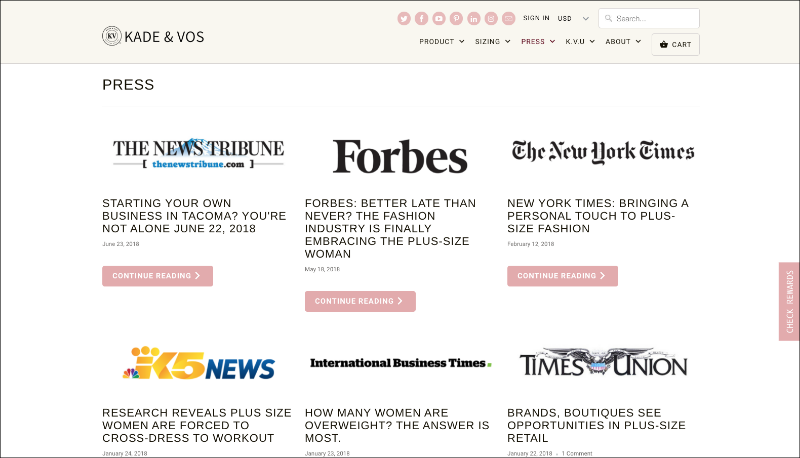Here is a cleaned-up and detailed caption for the image:

---

**Screenshot of Kade & Voss Website Interface**

In this screenshot of the Kade & Voss website, the top section features a light tan toolbar that spans the width of the page. On the right-hand side of the toolbar, there is a black circle with the initials "KV" in it, and the text “Kade & Voss” written beside in clear black ink. 

On the left-hand side of the toolbar, there are various social media icons, including Twitter, Facebook, Pinterest, Instagram, and YouTube, symbolizing easy access to their social media profiles. Additionally, there may be an email link and another unidentified icon. Further to the right, there are options for sign-in, selecting U.S. dollars as the currency, and a search bar.

Directly below the toolbar, you'll find a navigation menu with the following links: product sizing, press, KVU, about, and cart, indicating a user-friendly interface for those looking to shop or learn more about the brand.

The main screenshot displays a section titled “Press,” featuring six different articles. These articles highlight press coverage and fashion industry news related to plus-size fashion, suggesting that Kade & Voss is a brand that focuses on this market. The featured articles include:

1. **News Tribune**: "Starting your own business in Tacoma? You're not alone" (June 22, 2018). This article has a link labeled "Continue reading."

2. **Forbes**: "Better late than never? The fashion industry is finally embracing the plus-size woman."

3. **New York Times**: "Bringing a personal touch to plus-size fashion."

4. **K5 News**: "Research reveals plus-size women are forced to cross-dress to work out."

5. **International Business Times**: "How many women are overweight? The answer is most."

6. **Times Union**: "Brands, boutiques see opportunities in plus-size retail."

Each article preview is accompanied by a "Continue reading" link in pink. Additionally, a pink box in the middle left of the page says, "Check rewards." 

The diverse selection of articles and the user-friendly design elements such as "Continue reading" buttons and clear navigation suggest that Kade & Voss aims to provide an informative and accessible online shopping experience with a focus on plus-size fashion.